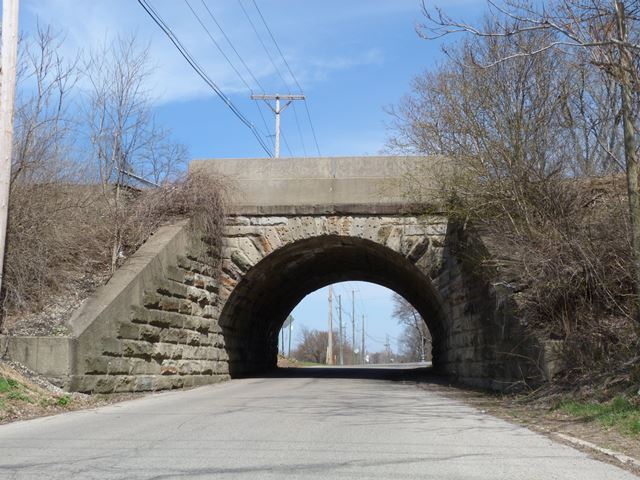This daytime color photograph captures a solitary road passing under an arched stone overpass. The overpass, possibly crafted from weathered stone or aged brick, stands prominently at the center of the image. The archway is dark inside, hinting at the tunnel’s depth and allowing a glimpse of the road continuing on the other side. A bundle of telephone wires stretches across the top of the frame, supported by unseen poles. To the right, a patch of green grass contrasts with the barren, leafless trees that suggest a wintry setting. On the left, a mix of dirt and rocks adds an earthy texture. The sky above is a serene blue, dotted with a few small white clouds, enhancing the crisp and clear day ambiance. The road itself is devoid of traffic or pedestrians, emphasizing the stillness and quiet of the scene.